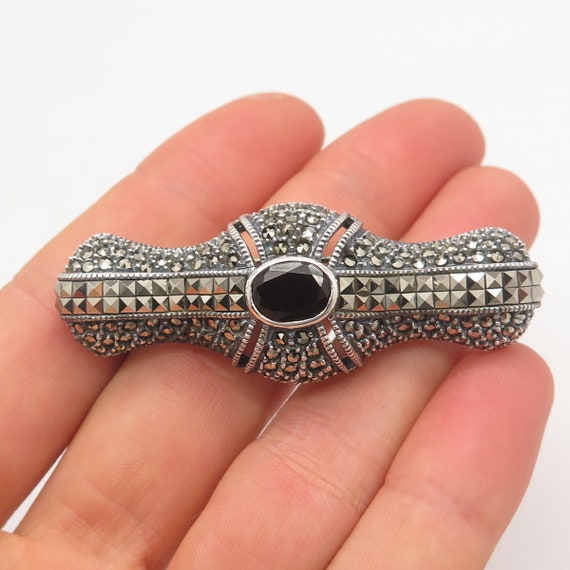The photograph captures a zoomed-in view of a light Caucasian European man's hand holding an intricately designed brooch. The hand, showing four fingers without the thumb, holds the item delicately in the fingertips. The brooch, lying horizontally across the fingers, spans their entire width. Its design features a distinctive shape, reminiscent of a pipe but with a unique, breadstick-like bulge in the center and narrowing at both ends, which resemble the ends of a pipe.

The brooch is adorned with a dazzling array of small silver gems and square jewels. Notably, a line of sparkling rhinestones extends through the center, accentuated by a prominent dark oval gem—a ruby—in the very middle. The design also includes two split areas in the center resembling backward parentheses, offering a glimpse of the hand beneath. The background of the image is pure white, emphasizing the hand and brooch’s intricate details. The overall aesthetic of the brooch suggests a piece of jewelry or a decorative hair accessory, like a barrette, made more striking by its elaborate craftsmanship.